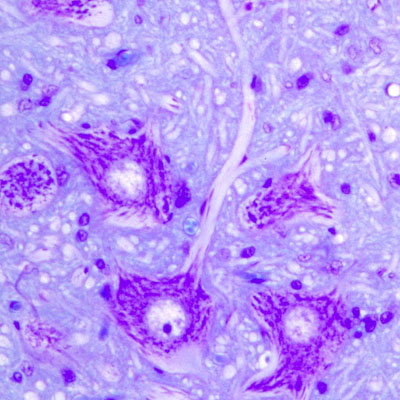This image is a highly magnified view of some kind of organism, likely captured through a microscope. The dominant color palette includes various shades of purple and blue, with the entire image enveloped in these hues, creating a somewhat monochromatic effect. Within this field, there are several larger, irregularly shaped dark purple circles, numbering around four to six, some of which appear cut off at the edge of the image. Notably, one of these larger circles features a distinctive white circle with a black dot in the center, resembling an eye, and has a light purple or white tail-like extension protruding from it. Scattered throughout the image are numerous smaller, darker purple splotches, devoid of any eye-like features, alongside tiny blue dots and light purple or white wisps that interlace the scene. The overall layout appears random and asymmetrical, with no obvious pattern, suggesting the natural randomness typical of microscopic organisms or cells.